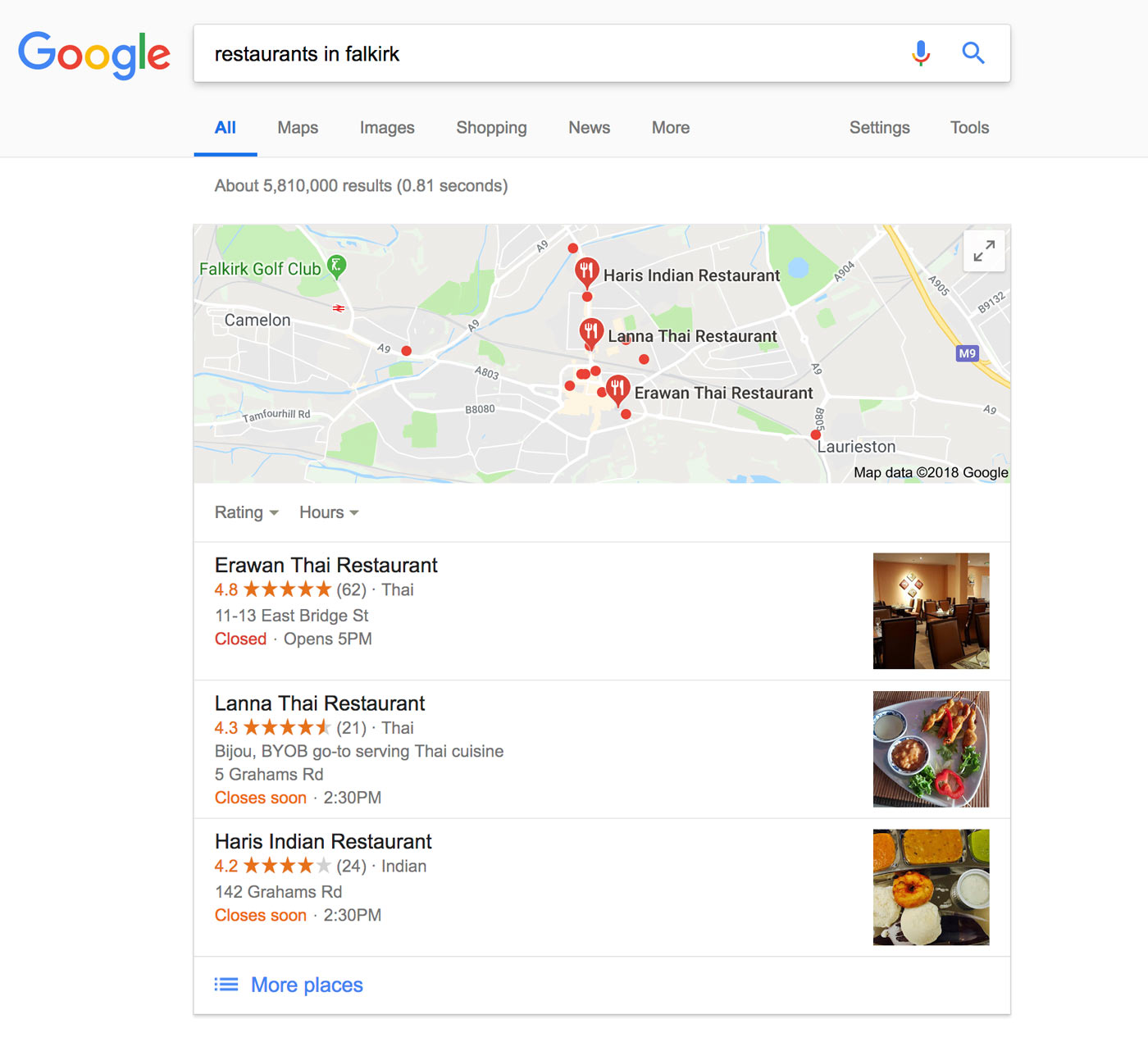The image captures a Google search results page displayed on a computer screen. At the top left corner of the page, the multi-colored Google logo is set on a very light grey background. Adjacent to the logo is a white text box containing the search query "restaurants in Falkirk," accompanied by a microphone icon and a magnifying glass icon on the right.

Directly below, in the grey menu bar, the clickable options include "All," "Maps," "Images," "Shopping," "News," and "More," with "All" highlighted in blue and underlined while the others remain in grey font. To the far right, options for "Settings" and "Tools" are visible.

Beneath this menu bar, on a white section of the page, is a grey line of text stating that there are about 5,810,000 results found in 0.81 seconds. Below this, a small map segment highlights three specific restaurants: Harris Indian Restaurant, Lana Thai Restaurant, and Erawan Thai Restaurant, along with several smaller red dots indicating additional restaurant locations.

Further down, detailed information about these three restaurants is listed, including their ratings and contact details. Erawan Thai Restaurant is listed first with a rating of 4.8 stars, followed by Lana Thai Restaurant with a 4.3-star rating, and Harris Indian Restaurant with a rating of 4.2 stars.